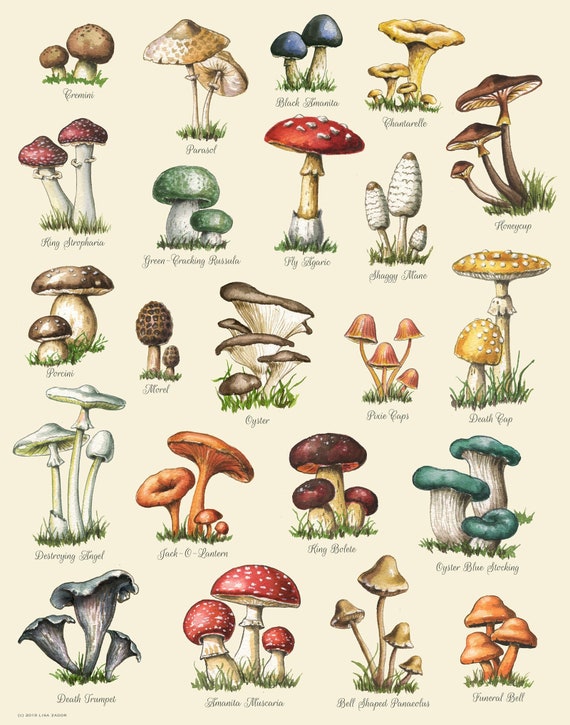This poster features a beautifully illustrated collection of various mushroom types against a tan and whitish background. Each mushroom illustration is colorful, whimsical, and detailed, with textures that bring the fungi to life. The poster includes around 20 different types of mushrooms, such as creminis, chanterelles, morels, porcinis, death caps, oyster blues, jack-o'-lantern mushrooms, destroying angel, death trumpet, and funeral buff. Each type is accompanied by neatly spaced illustrations of multiple mushrooms, often two or more per type, emerging from patches of grass. The mushrooms display a palette ranging from brown, blue, red, green, orange, yellow, to dark brown and teal blue, with some featuring polka dots or small white areas on their caps. Fancy script labels beneath each mushroom enhance the poster, although the text is quite small and intricate. This poster serves not only as a charming piece of art but also as an informative infographic, clearly distinguishing the varied characteristics and appearances of each mushroom through well-organized visuals and descriptive labels.